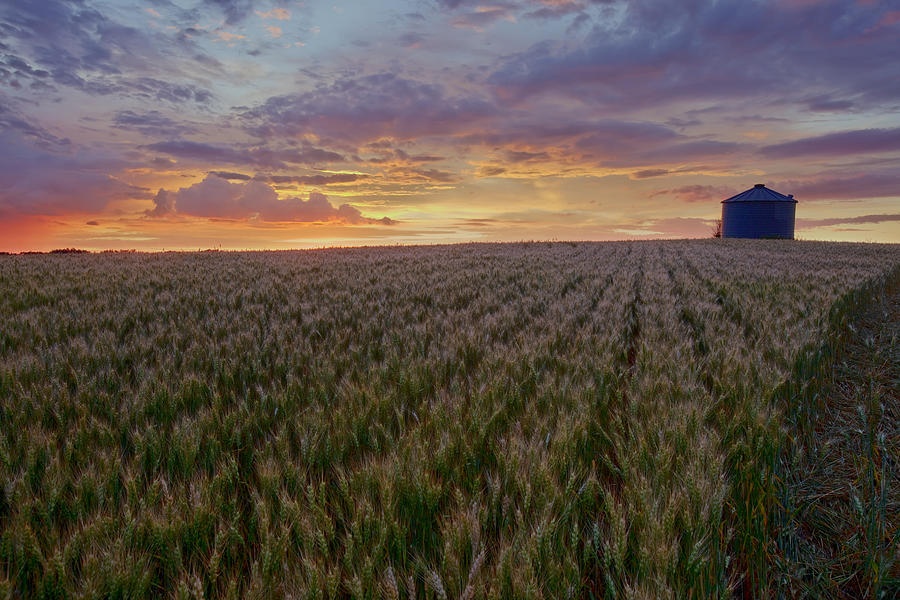The photograph captures an expansive wheat field that seems to stretch endlessly into the horizon, characterized by neatly aligned rows. Near the edge of the field, a barn and a cylindrical silo capped with a cone-shaped roof are visible, indicating that this is an active farmland. The sky is a stunning tapestry of colors, indicative of a beautiful sunset. The lower part of the sky glows with deep orange and yellow hues, transitioning to softer shades of pink and peach, and finally merging into a serene blue as it ascends. Numerous clouds, varying from white to gray, add texture to the vibrant sky. The overall scene evokes a serene and picturesque rural landscape at twilight.